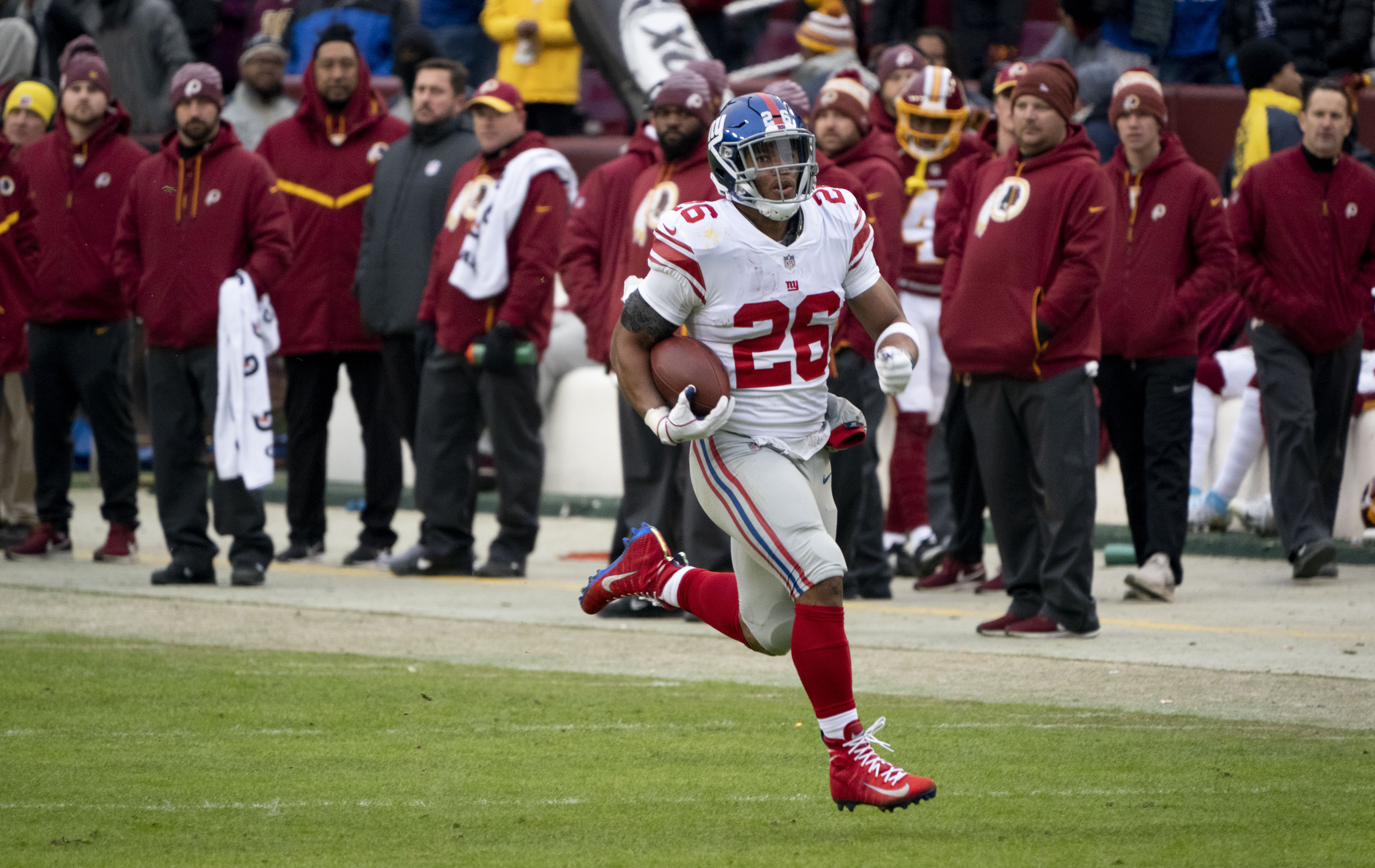This detailed photograph captures an African-American football player mid-run, clutching a football securely in his right arm. He is dressed in a white football uniform that includes a white jersey emblazoned with the red number 26 on the front, back, and shoulders. He sports light gray pants, adorned with two red and one blue stripe running vertically down each side. His ensemble also features a navy blue helmet with white text and a red stripe, red Nike cleats with white laces, long red socks, and white gloves.

In the background, spectators are either seated or standing, sporting dark red or burgundy attire with some yellow accents, and some are donning hats or holding towels. The grassy field beneath the player is green, with faded white lines marking the play area, adding to the dynamic atmosphere of the football game being captured.